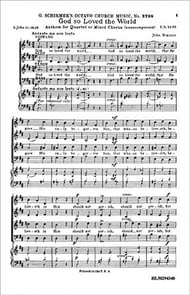The image depicts a page from a hymnal, specifically showcasing sheet music for a well-known Christian classical song titled "God So Loved the World" by composer John Stainer. The sheet is white with intricate black music notation. Though the print is small and some text is blurry, the title at the top is clearly legible. This page is one of four, and it is designed for a mixed choir, often performed a capella. The sheet music is divided into 18 lines of notes, arranged in three sets of six, which likely correspond to different parts of the song, including verses and possibly the chorus. The piece is published by G. Schirmer in an Octavio format, providing detailed musical guidance that would be familiar to those adept at reading sheet music.